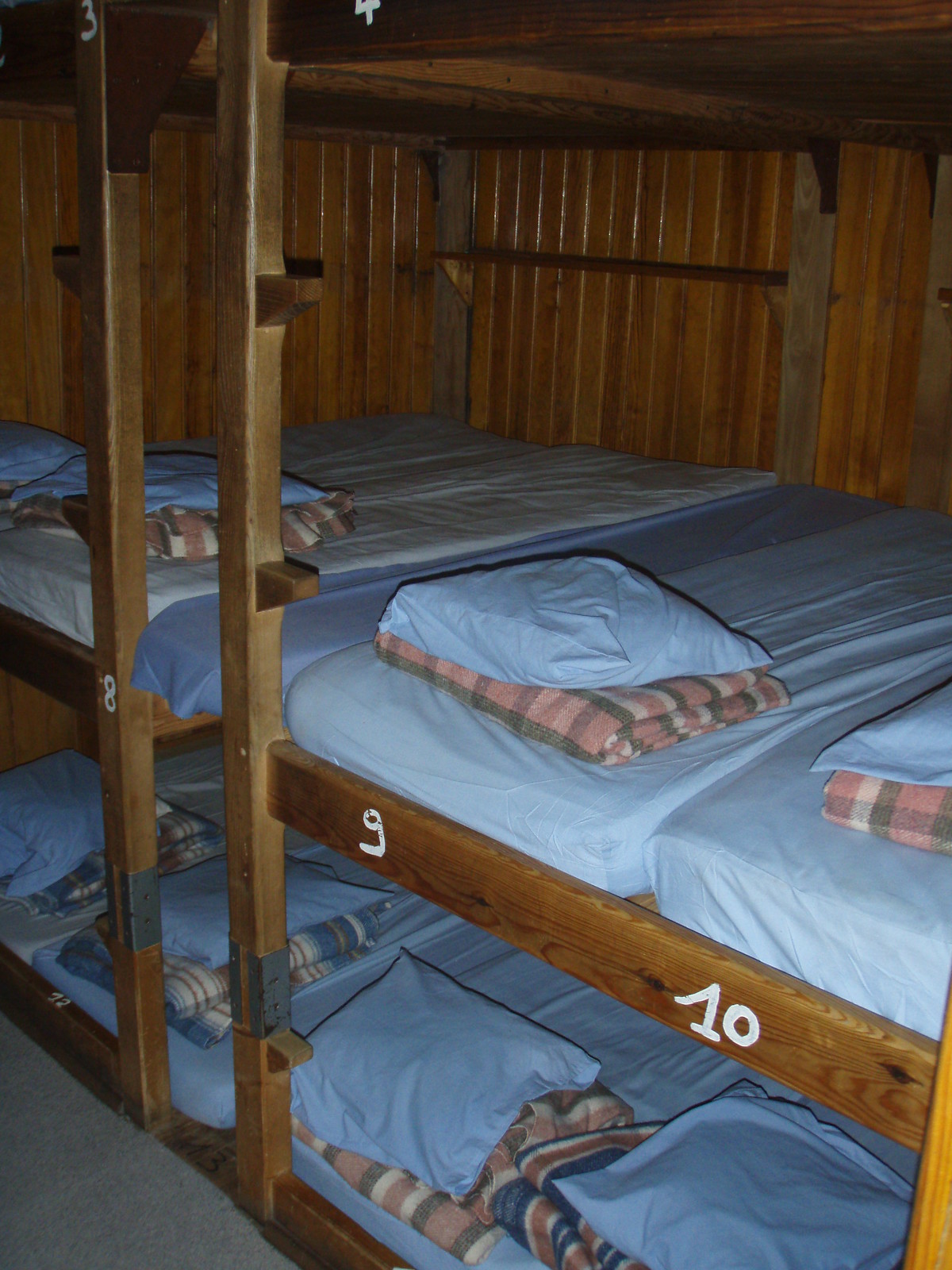The color photograph showcases the interior of a rustic wooden cabin that seems to be part of a summer camp or similar communal sleeping quarters. The room features multiple bunk beds with glossy red oak frames, arranged diagonally from the center left to the bottom right of the image. Each bunk bed stack appears to be a triple-decker design, with visible beds labeled with hand-painted white numbers 8, 9, and 10 on the wooden frame. The bunk beds are tightly packed, creating a cramped appearance reminiscent of old-style barracks.

Each twin-sized mattress is dressed in a light blue sheet, complemented by a matching blue pillow. A plaid or striped blanket, featuring colors like pink, green, white, and blue, is neatly folded atop each mattress. The beds are stacked so closely that the space between levels is notably narrow, and the wooden support beams indicate potential for additional bunks to be added. The photograph also captures the cozy ambiance of the cabin, complete with wood-paneled walls and a visible section of grey flooring in the bottom left corner. Overall, the image evokes a sense of shared camaraderie and practical functionality typical of group camping experiences.